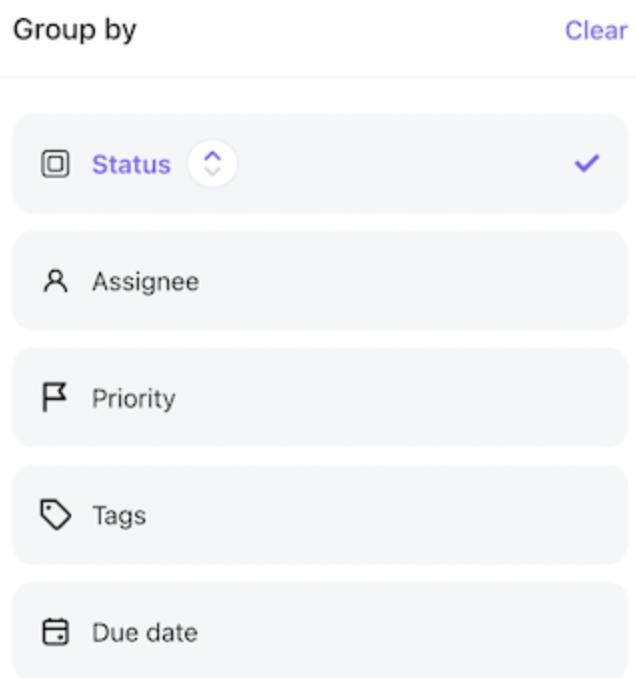The top left corner of the image features the text “Group By” in black, while the top right corner displays the word “Clear” in blue. Below these words, a thin gray line spans the width of the image. 

Beneath this line, the white background houses five distinct fields, each represented by a gray, rounded rectangle button with specific labels and icons. 

1. The top field is labeled “Status” in blue text. It includes a symbol featuring a white circle with a blue upward arrow and a gray downward arrow. On its left, there is an icon resembling two overlapping squares, and on its right, a blue checkmark.
2. The second field, “Assignee,” shows an icon of a person.
3. The third field, labeled “Priority,” has an icon of a black flag.
4. The fourth field, “Tags,” displays a black price tag icon.
5. The fifth and final field, “Due Date,” includes a calendar icon to its left. 

Each field provides a clickable button designed with functionality in mind, making the interface organized and user-friendly.